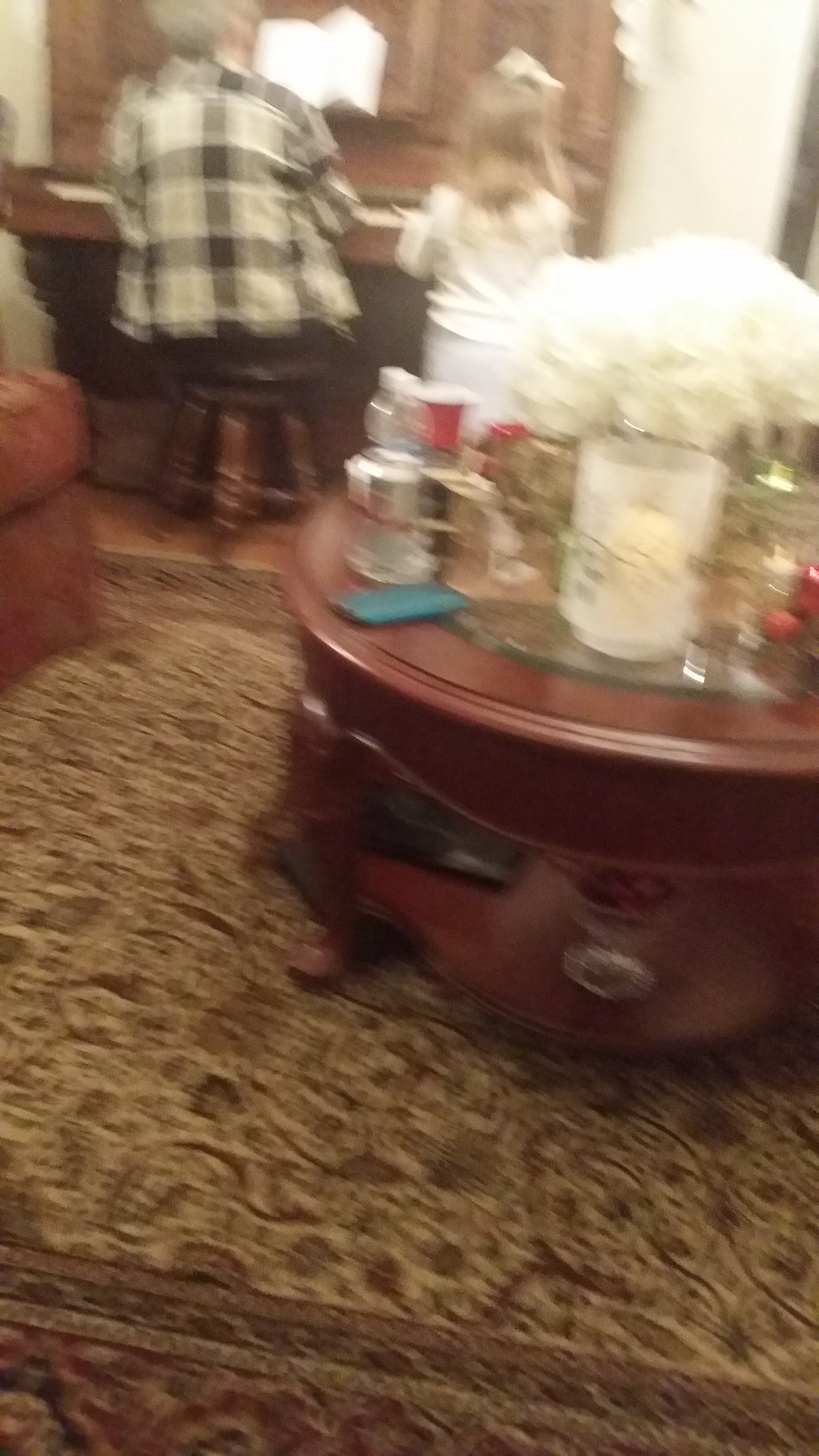The photograph, presented in color and portrait orientation, captures a cozy, albeit cluttered, living space. The foreground features an intricately patterned oriental rug in shades of tan, maroon, and brown, partially obscured by a round cherry wood coffee table. The table itself is laden with various objects, including a visible soda can. Slightly further back, a rust-colored recliner adds warmth to the scene.

In the background, attention draws to a young blonde girl with white-blonde hair, standing beside a wooden piano. Seated at a stool next to her is a woman with silver hair, dressed in a black-and-white checkered shirt. She appears to be instructing the child, as evidenced by the open songbook in front of her. The overall ambiance is one of familial intimacy and learning, marred only by the photo's blurriness, particularly noticeable in the distant parts of the image.